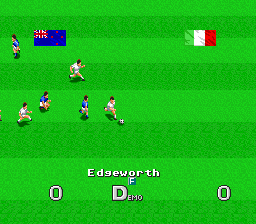In this small, pixelated screenshot of an old soccer-themed video game, likely from the 80s or 90s, we see a vibrant depiction of an in-game soccer match. The green field, adorned with alternating light and dark green stripes simulating freshly cut grass, sets the stage. Six players are visible: three in blue uniforms and three in white uniforms and shorts, all seemingly in motion, chasing a black and white soccer ball. Shadows cast by the players add a touch of depth to the low-resolution graphics. In the top left corner, an Australian flag is visible, while an Italian flag occupies the top right corner. The bottom of the image features a scoreboard displaying a 0-0 score, and in the center, the word "Demo" is prominently displayed. Additionally, the name "Edgeworth F." suggests a player's identity, likely a forward position, indicated on the screen.